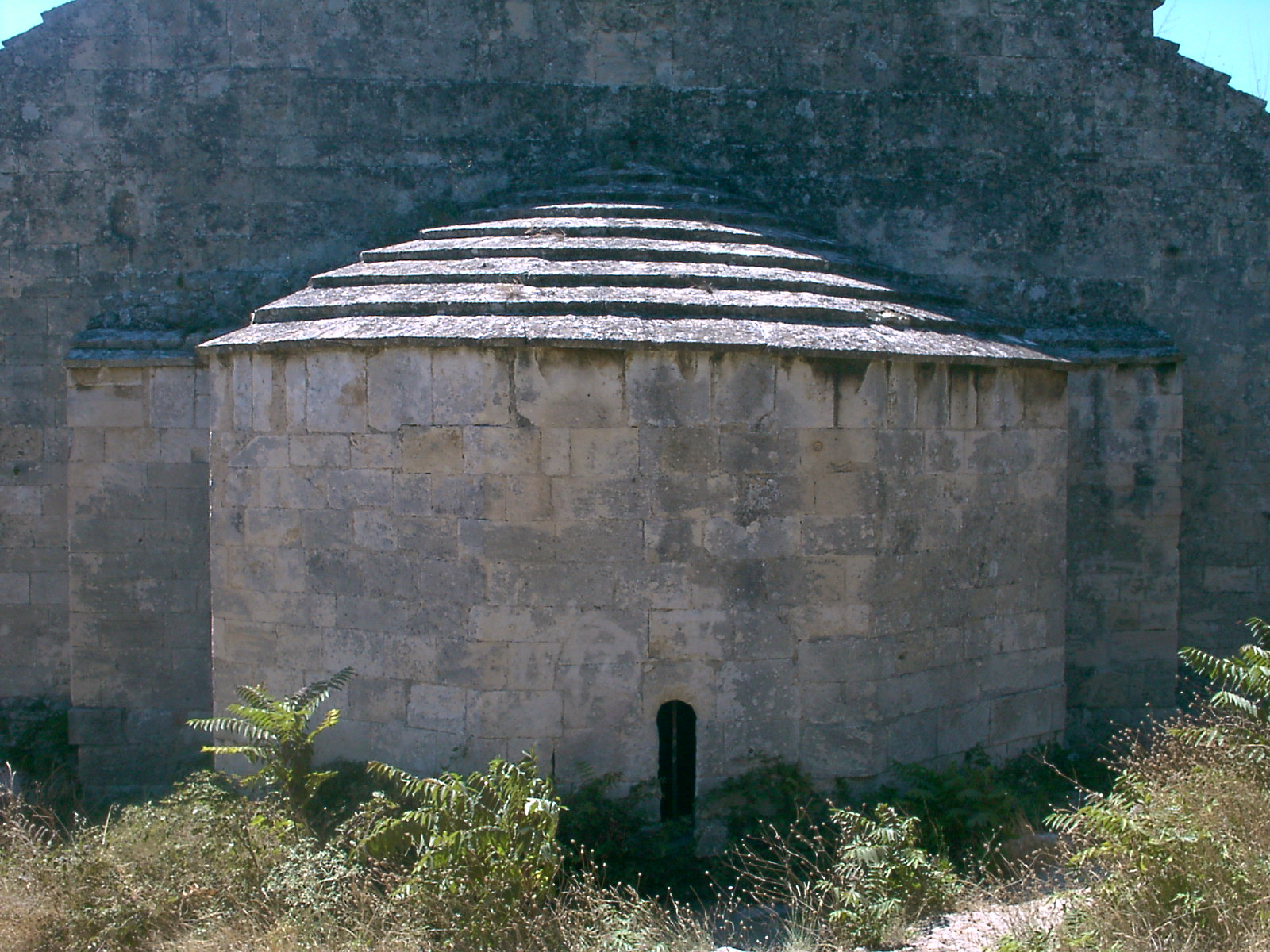In the photograph captured outdoors during the daytime, a historical stone structure dominates the scene. The image, wider than it is tall, frames a stretch of old stone wall that spans the width of the photo, reaching down about four-fifths of the way from the top. In the upper corners, patches of blue sky peek through, adding a touch of calmness above the ruggedness below. 

Approximately a quarter of the way down the image, an architectural extrusion emerges from the wall. This structure features a rounded, silo-like form with a distinctive roof composed of narrow, tiered steps that flare out at the base, resembling a series of graded shingles. This rounded section is constructed entirely from gray stone and has an aged, weathered appearance. 

Directly beneath the eaves of the roof, discoloration suggests moss or water damage, emphasizing the structure's antiquity. At the very bottom center of this rounded extrusion, there is a narrow, oval-shaped entrance, akin to a medieval castle's doorway, hinting at a dark, possibly unused interior. This entrance adds an air of mystery to the scene, evoking thoughts of secret passages or forgotten chambers.

On either side of this central rounded structure, smaller rectangular stone constructions flank it, enhancing its prominence. The base of the scene is enveloped in lush, overgrown green brush interspersed with patches of white sand, hinting at neglect and the persistence of nature. Additionally, in the bottom right corner, a small dirt pathway meanders, possibly suggesting former human activity. The sunlight casts bright highlights on the plants and the weathered stone surfaces, adding depth and character to the timeless tableau.